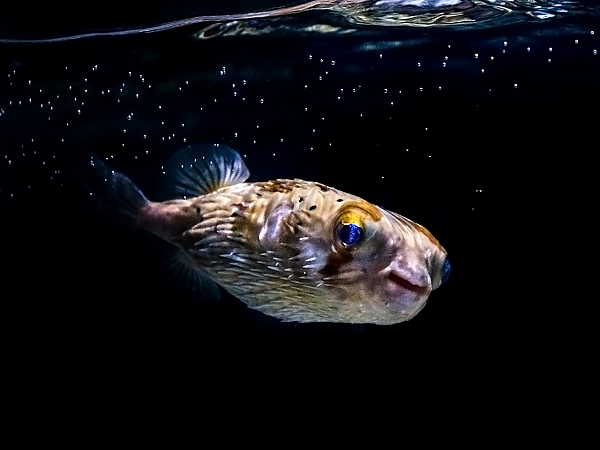The image depicts a baby puffer fish, also known as a porcupine fish, against a dark, aquarium-like background. The water is clear and well-lit, with slight spots below indicating bubbles or water patterns. The fish itself is vividly colorful: it has big blue eyes with hints of orange or yellow around the eyelids, giving it an almost smiling appearance. Its body is round and chubby, primarily purplish around the mouth and belly, transitioning to brownish and tan hues towards the back, accented with darker and white spots. The spines lie flat against its body, adding to its endearing, cute look as it swims in the clear black water.